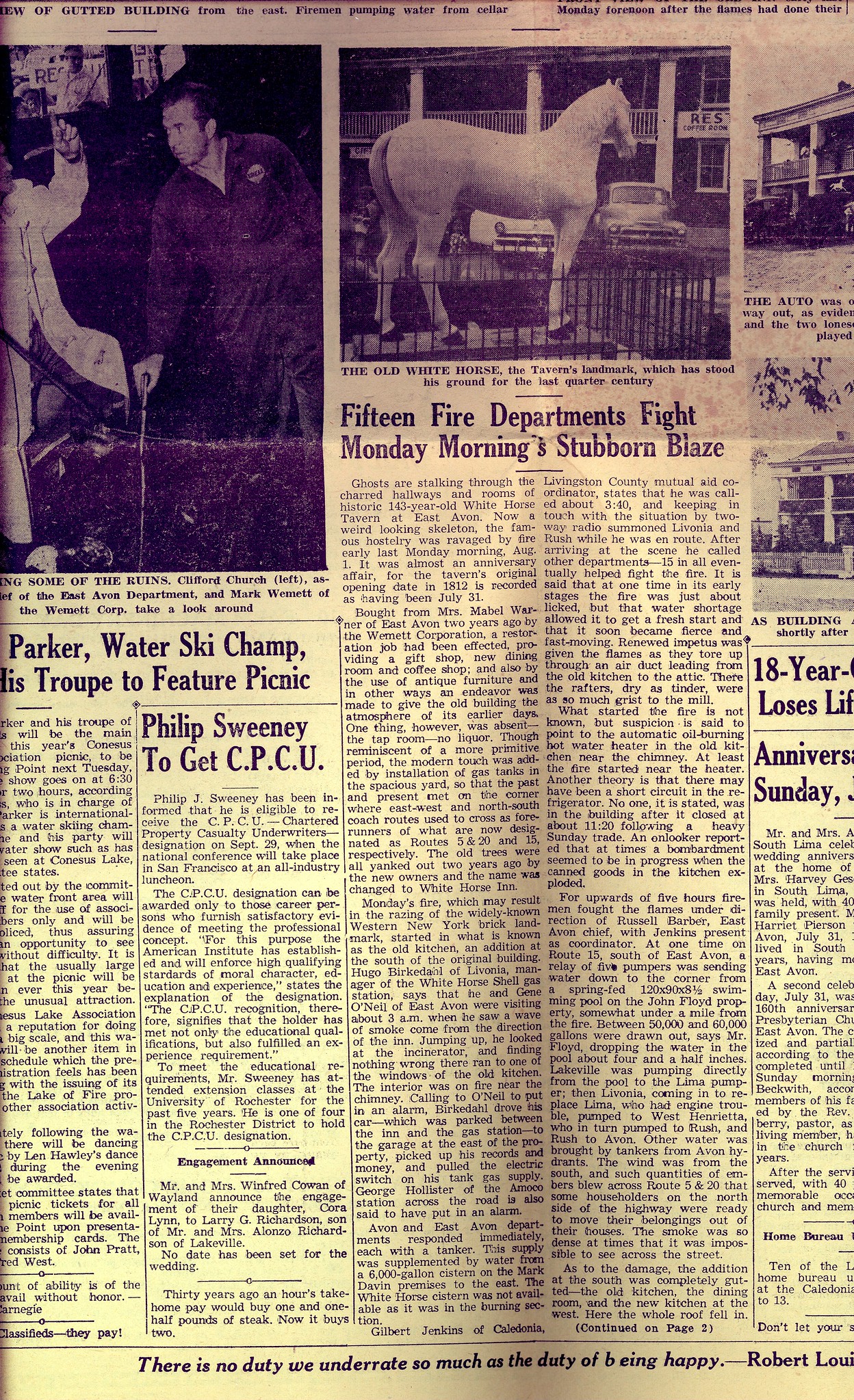This image depicts a long, yellowed, vertical rectangle-shaped newspaper page, giving off a distinctly aged and weathered appearance. The newspaper appears to be quite old, possibly from the 1950s. It is filled with numerous articles and headlines, each crammed in typical fashion for that era. 

Prominently, at the top of the page, there are three black-and-white photographs. The left-most photograph shows two men, one of whom is holding a cane, identified as Clifford Church of the East Avon Department and Mark Wemmett of the Wemmett Corp. The center photograph features a man in coveralls alongside another in a white lab jacket. The third photograph displays a white horse statue surrounded by a black railing, referred to as the old white horse, a tavern landmark that has stood its ground for the last quarter of a century.

Numerous articles headline the page, notably one about a stubborn blaze fought by 15 fire departments on Monday morning at the historic 143-year-old White Horse Tavern in East Avon, which suffered significant fire damage on August 1st. Another prominent article discusses Parker, a water ski champion, and Philip Sweeney, who is to receive a CPCU, suggesting a celebratory tone. The overall layout is dense with descriptive text and historical imagery, capturing a slice of a bygone era.